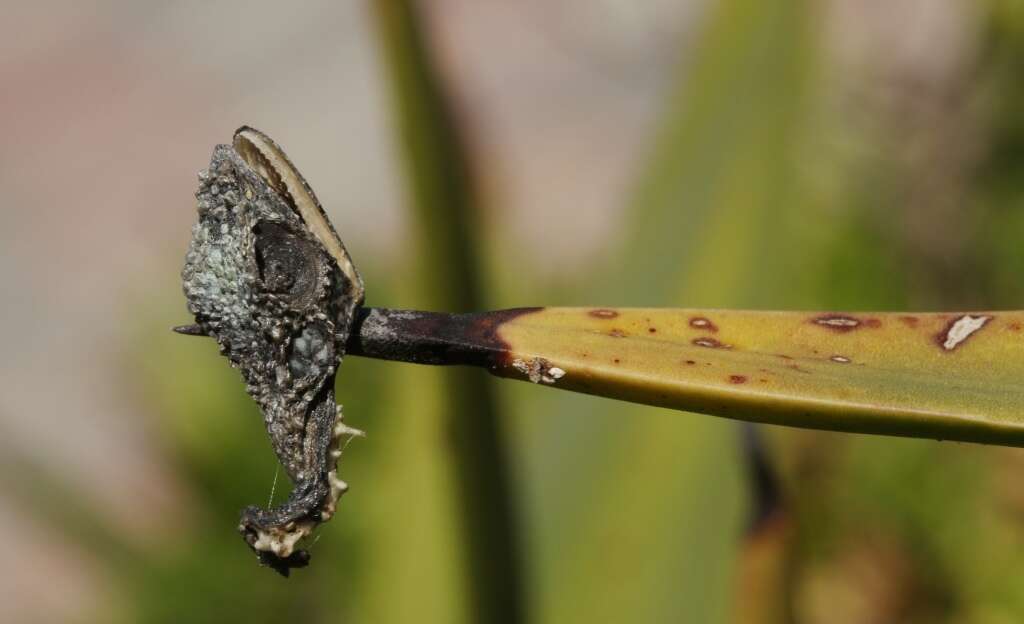The photograph captures an outdoor scene with a blurred, green and brownish-gray background of vegetation. In the foreground, a green leaf with reddish-brown spots and a sharply pointed tip extends from the right side of the image toward the left. The tip, appearing black, seems charred or degraded. At this blackened edge, there is an intriguing structure resembling the head of a small lizard or reptile. The head, which is gray and scaly, faces upwards with the back towards the camera, showing a slightly open mouth with tiny teeth, a small eye, and distinct scales. The description also suggests an alternative interpretation of the structure as a cocoon-like pupa, characterized by its diamond-shaped form with a split top, displaying black and light blue hues.